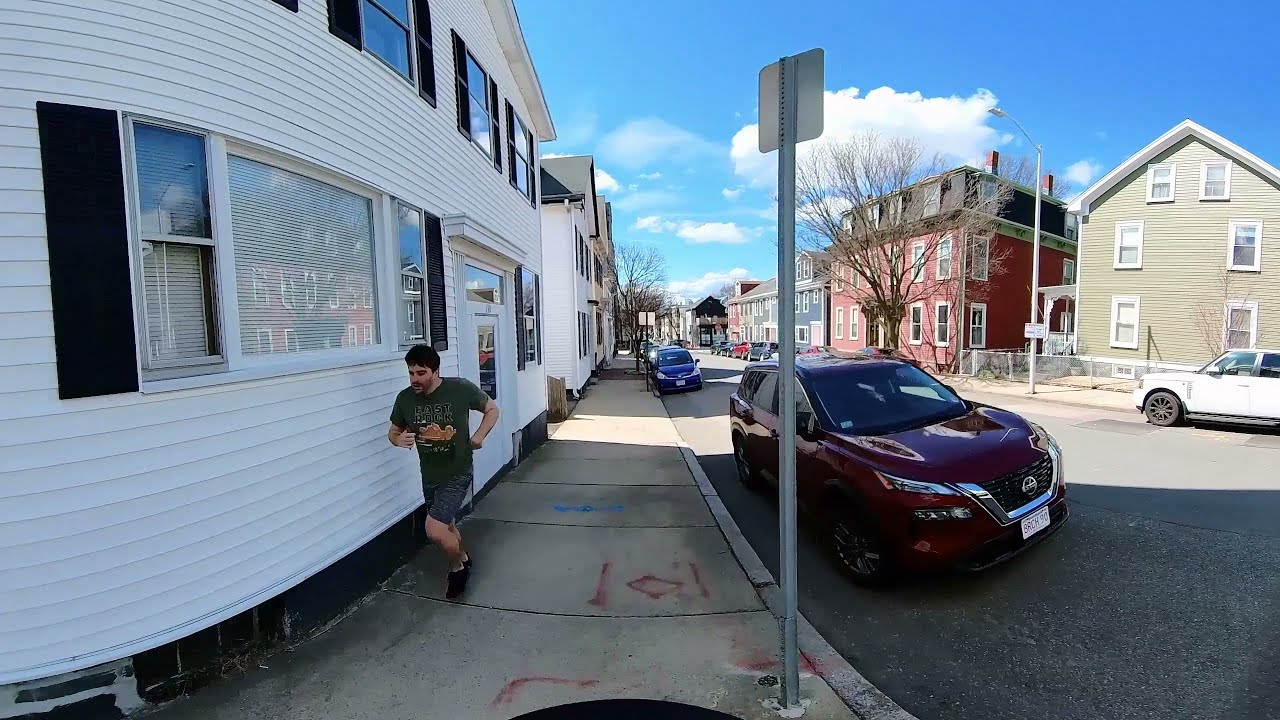In this detailed daytime photograph, a man with short black hair and a five o'clock shadow is depicted running towards the camera along a sidewalk. He is dressed in a dark green t-shirt, which has an indistinguishable image on the front, dark gray shorts, and black shoes. The sidewalk he’s running on is gray and shows remnants of both blue and red spray paint, including a diamond shape outlined in red lines near the front of the image.

To the left of the image is a row of white, two-story buildings, likely houses, accentuated with black trimmed windows and black shutters. On the right side of the sidewalk, parked along the curb, is a dark maroon SUV, partially in shadow. Further down the street on the right side, additional cars can be seen, including a white vehicle in front of one of the homes.

The background showcases more homes on the opposite side of the street, varying in color and height. Prominently, there is a three-story red building adjacent to a tan building with white window borders, and further along, a blue house as well as another red structure. The scene is enriched by leafless trees, pointing towards a winter season, under a blue sky dotted sparsely with white clouds, establishing a serene neighborhood setting.